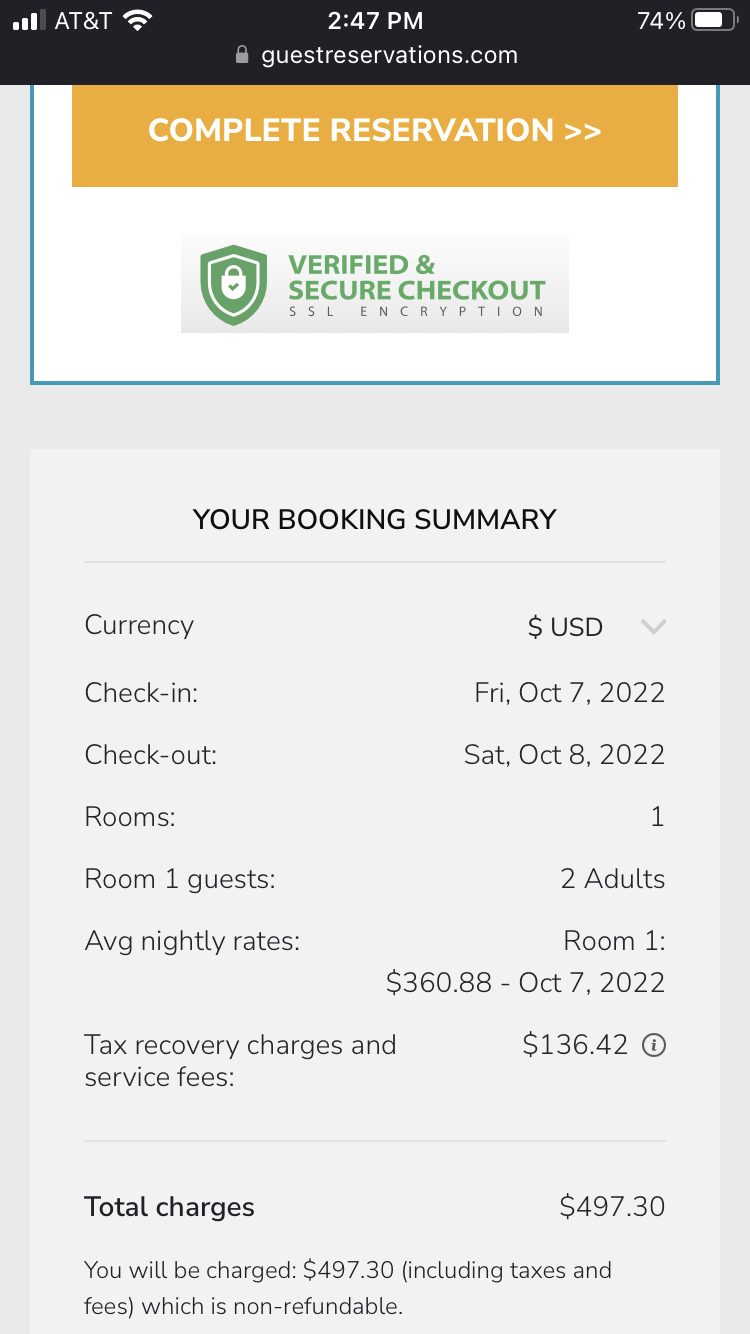A screenshot of a mobile phone displays several details. In the top right corner, the status bar indicates a cellular connection with three out of four bars, AT&T as the carrier, a time of 2:47 p.m., and a battery life at 74%. Beneath the status bar, the screen shows a message indicating a secure connection to guestreservations.com.

The middle section of the screenshot features a partially visible gold rectangle button labeled "Complete Reservation" and a green shield icon with a lock, signifying verified and secure checkout with SSL encryption. All this information is contained within a white rectangle with blue trim.

The lower section of the screen provides a summary of the booking details. The booking is in U.S. dollars, with check-in on Friday, October 7th, 2022, and check-out on Saturday, October 8th, 2022, for one room accommodating two adults. The average nightly rate for the room is listed as $360.88. Additional charges include tax recovery fees and service charges amounting to $136.42. The total cost for the booking is $497.30, which is non-refundable and will be charged to the user.